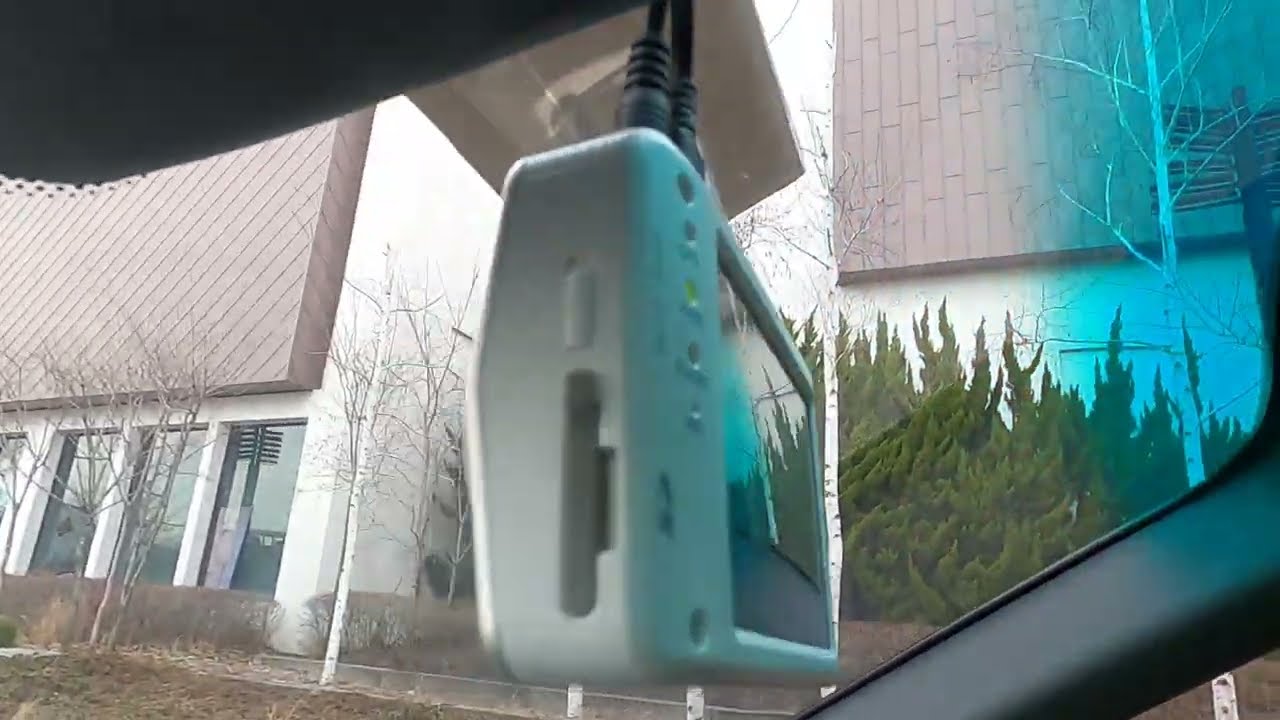The image captures the interior of a vehicle, providing a side view of a mounted GPS device with a white frame and screen. The close-up shot is somewhat blurry, revealing five indicator lights on the side of the device, with one lit up green. The device, resembling a GoPro or walkie-talkie, reflects the exterior scene on its screen. Outside the car windshield, two distinct buildings can be seen. These buildings, with brown brick roofs, are separated by a distance and surrounded by numerous tall, green plants and some dry trees along the sidewalk. The white buildings and lush greenery outside the vehicle are in sharper focus compared to the device, emphasizing the exterior scenery over the interior details.